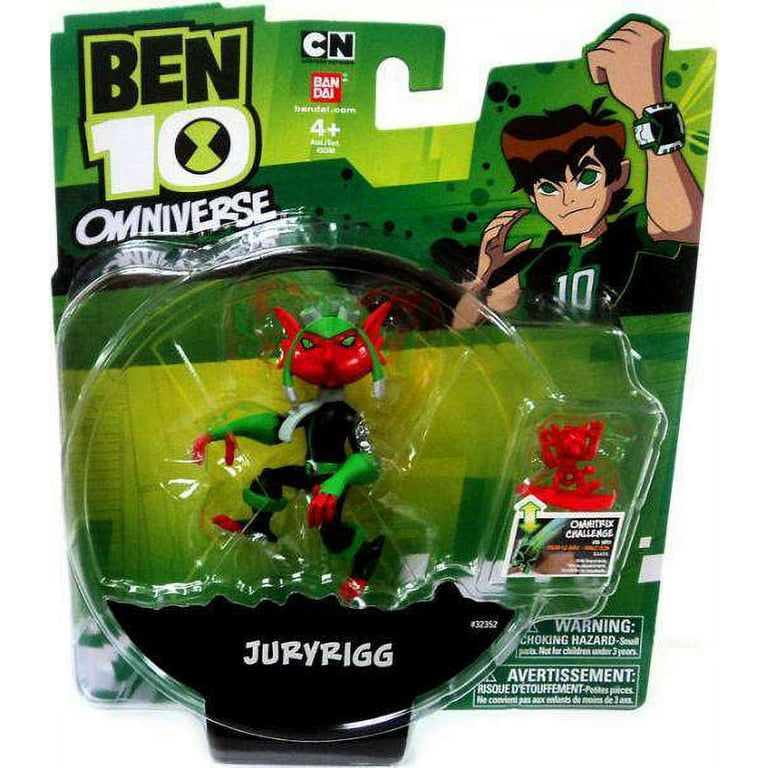This is an image of a Ben 10 Omniverse toy package against a plain white background. The package predominantly features green coloring with a thin plastic cover encasing the toy. In the top left corner, the package displays the Ben 10 Omniverse logo, accompanied by the Cartoon Network logo and another logo that appears to say Bandai, although the A's are styled as triangles. Indicated for ages 4 and up, the package includes a choking hazard warning at the bottom right. The toy, named Jury Rig, is presented within the package. The action figure is designed with a red head and ears, green eyes, and a green helmet-like feature covering its head. It has black attire with a belt featuring a silver buckle, red hands, red feet, green sleeves, and a green-and-black uniform. Additionally, the toy includes a smaller red mini-figure labeled as an Omnitrex challenge. There is also an illustration of a cartoon boy in the upper right corner of the packaging.